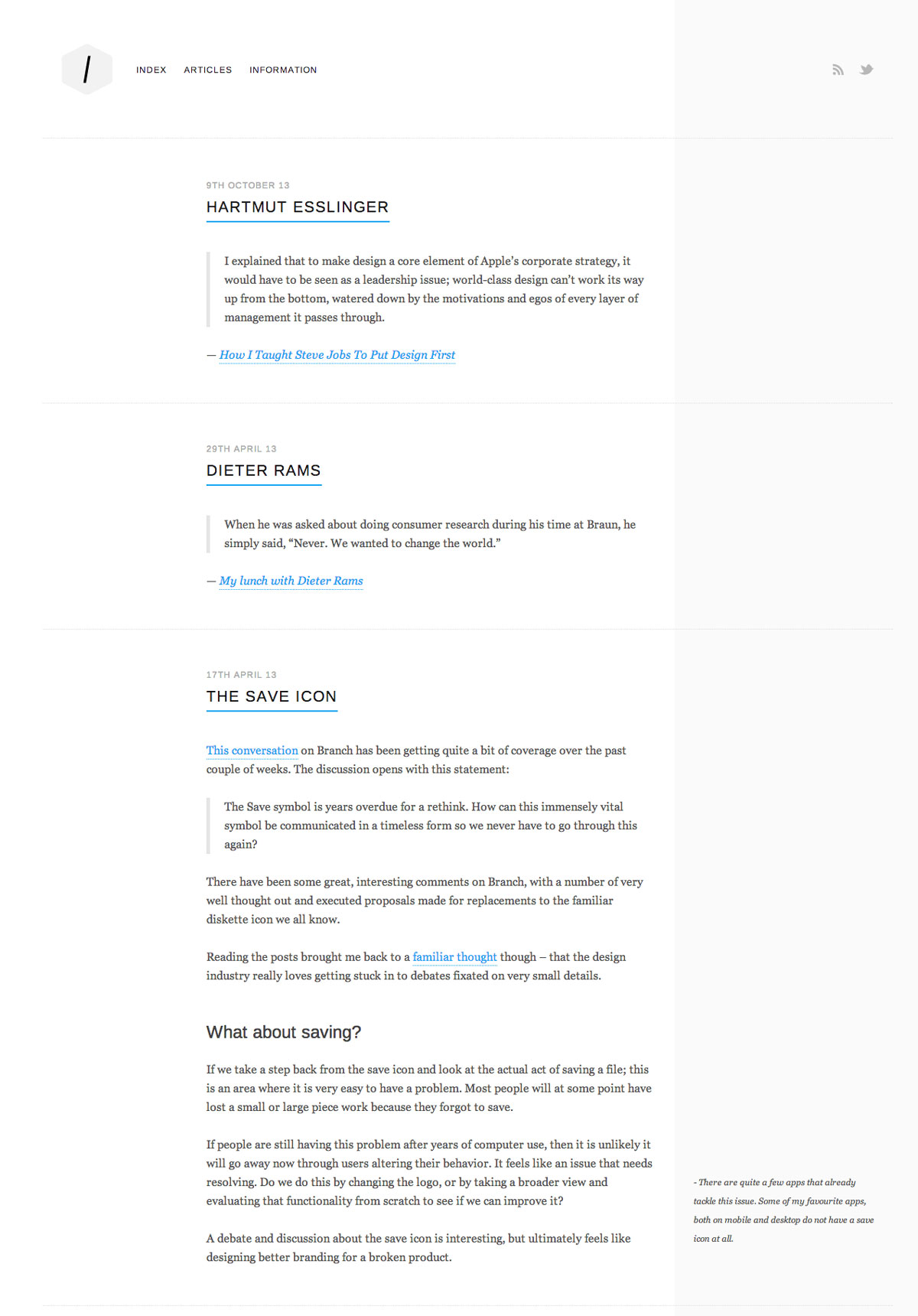The image displays a collection of posted articles. At the very top, there is a grey hexagon containing the letter "I," symbolizing information. Next to this icon are the words: "Index," "Articles," and "Information," with a Twitter link located on the far right. 

Beneath these headings, a series of articles from various dates are listed. The first article, published on October 8, 2013, is titled "Hartmut Esslinger." It discusses Apple's corporate strategy, specifically how Hartmut Esslinger influenced Steve Jobs to prioritize design. 

The second article, dated April 29, 2013, is called "Dieter Rams" and recounts a lunch meeting with the famous designer Dieter Rams. 

The third article, published on April 17, 2013, is titled "The Sea of Icons," which explores the potential need for updating and rethinking the long-used symbol. 

Each article delves into different aspects of design and its impact on technology and corporate strategy.